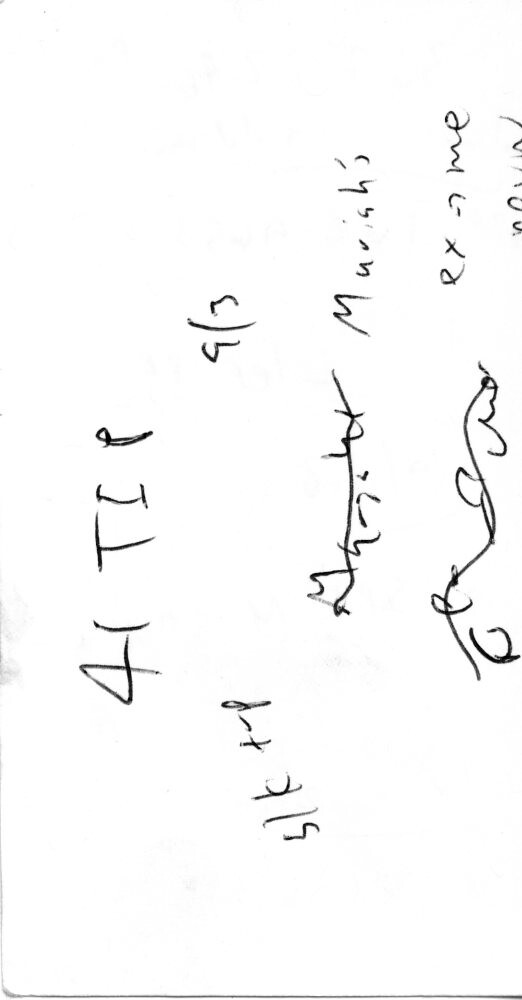The image showcases a sideways photograph or photocopy of a piece of paper filled with handwritten notes. The text on the paper is difficult to decipher, with several lines of writing that seem cryptic or fragmented. At the top of the paper, the phrase "for I tip" is barely legible, followed by a notation "9/3." Below this, another line reads "5 L K T - P," suggesting the possibility of a math problem, personal notes, or financial records. Additional writing can be seen on the paper, but it remains mostly illegible, obscuring the overall purpose or context of the document. The orientation and the ambiguous content of the writing contribute to the overall mystery of the notes' intent or meaning.